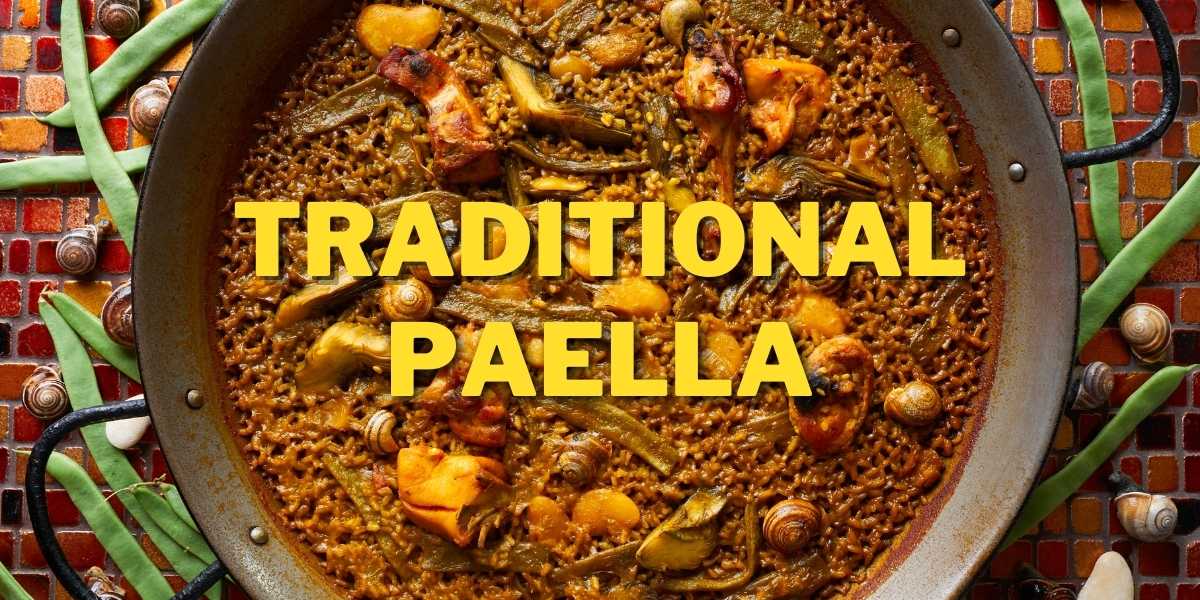The image showcases a large, shallow brown pot, possibly made of cast iron or copper, filled with traditional Spanish paella. The paella is a hearty mix featuring chunks of meat, green beans, peas, and snail shells. The pot, with black metal handles, takes up most of the rectangular photograph, which seems to be intended for a website or video thumbnail. Across the middle of the pot, in large yellow capital letters, the text "TRADITIONAL PAELLA" stands out prominently. The pot is set on a surface made of small, earth-toned, red and yellow tiles with gray grout. Scattered around the pot for a decorative touch are bright green, uncooked green bean pods, and additional snail shells, enhancing the overall rustic and traditional presentation of the dish.